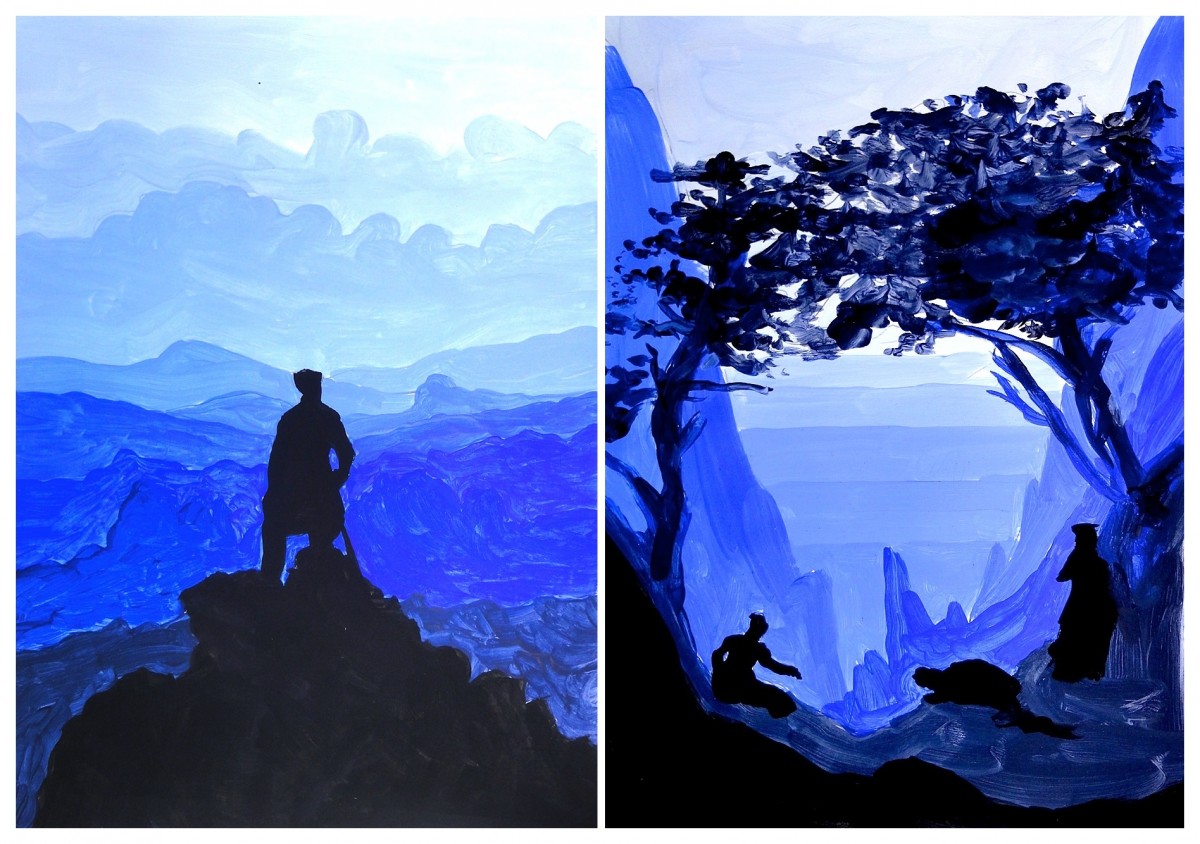The image features two distinct exterior scenes, each rendered in a painting or graphic style without any text, placed side by side in portrait mode. Both images are characterized by layers of silhouettes and evoke a serene, contemplative atmosphere.

**Left Panel:** This scene depicts the silhouette of a lone figure, possibly a man, standing on the edge of a hill or cliff. He appears to be wearing a long robe, facing away from the viewer, and his right leg is raised, perhaps resting on a stone. The cliff and the figure are entirely in black silhouette, creating a striking contrast against the layered backdrop of mountains. The mountains transition from dark blue in the foreground to light blue as they recede into the background. Above, the sky is filled with clouds that grow lighter and whiter as they rise, adding to the sense of depth and scale in the painting.

**Right Panel:** This image is set in a valley or ravine, featuring a trio of human silhouettes. On the left, a seated figure extends an arm towards a large turtle perched on a nearby cliff. To the right of this figure, another individual is kneeling, possibly in a prayerful pose, while a third person stands further to the right, leaning against the cliff. These figures are all rendered in black silhouette. Above them, two trees create a natural canopy, and the scene extends into a background of blue cliffs forming the sides of the valley. The cliffs descend into smaller protrusions like little towers, converging towards a vanishing point with a white sky and increasingly darker blue bands.

Both paintings use a minimalist, yet evocative color palette of blues and blacks to contrast the sharply defined silhouettes against a hazy, ethereal landscape.